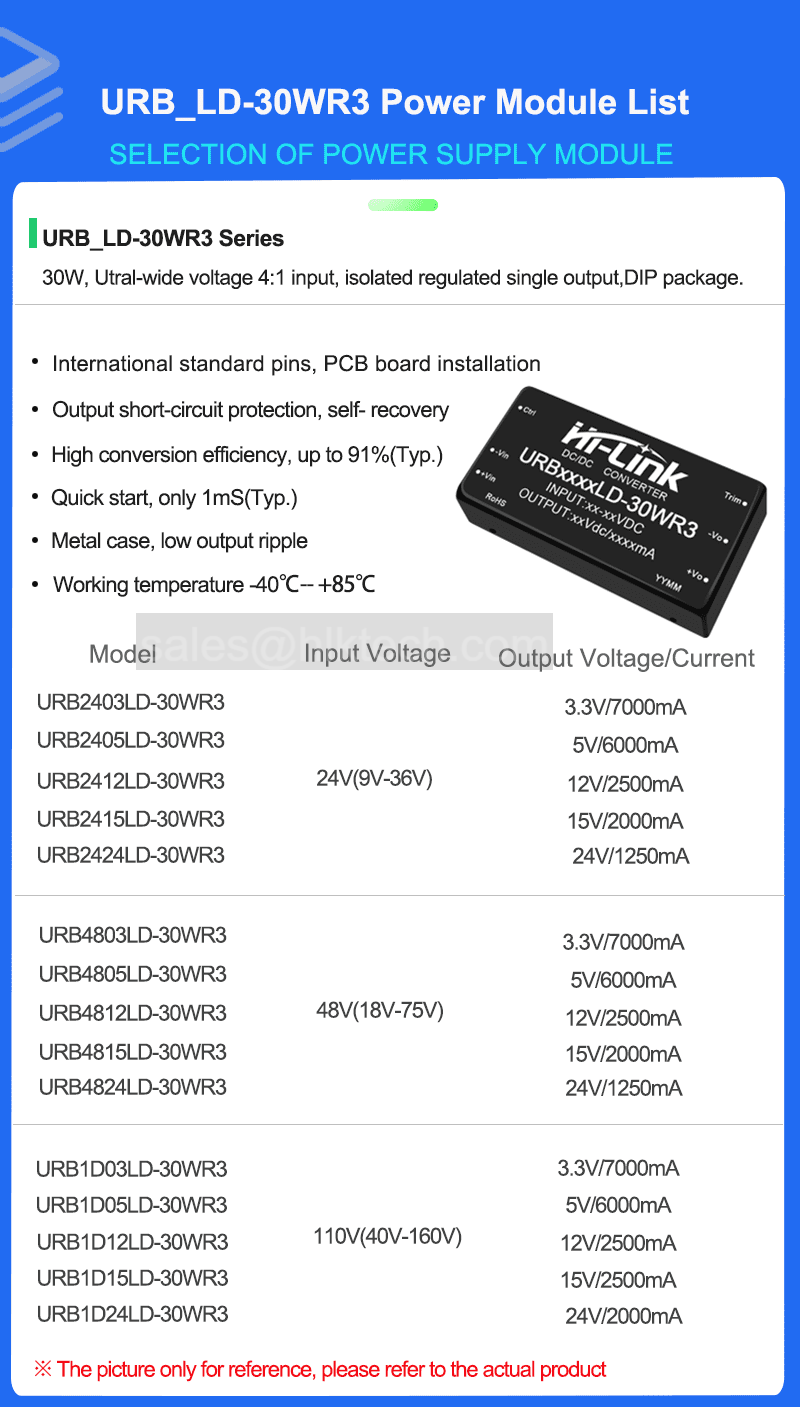A mobile phone screen displaying a web page with detailed information about a power module. The web page features a blue border with white and sky-blue text, and a white central area. The text within the blue border reads "URB_LD-30WR3 Power Module List" in white and sky-blue. In the white section, prominent black text reads "URB_LD-30WR3 Series" followed by "30 W Ultra Wide Voltage 4:1 Ratio Input Isolated Regulated Single Output DIP Package." 

Below the descriptive text, an image of the power module is displayed, accompanied by bullet points highlighting key features:
- International standard pins
- PCB board installation
- Output short circuit protection with self-recovery
- High conversion efficiency up to 91% TYP
- Quick start: only 1 ms TYP
- Metal case with low output ripple
- Operating temperature range: -40°C to +85°C.

Additionally, the same model’s output voltage and current specifications are listed. At the bottom, there is a red disclaimer text that states, "The picture is only for reference, please refer to the actual product."